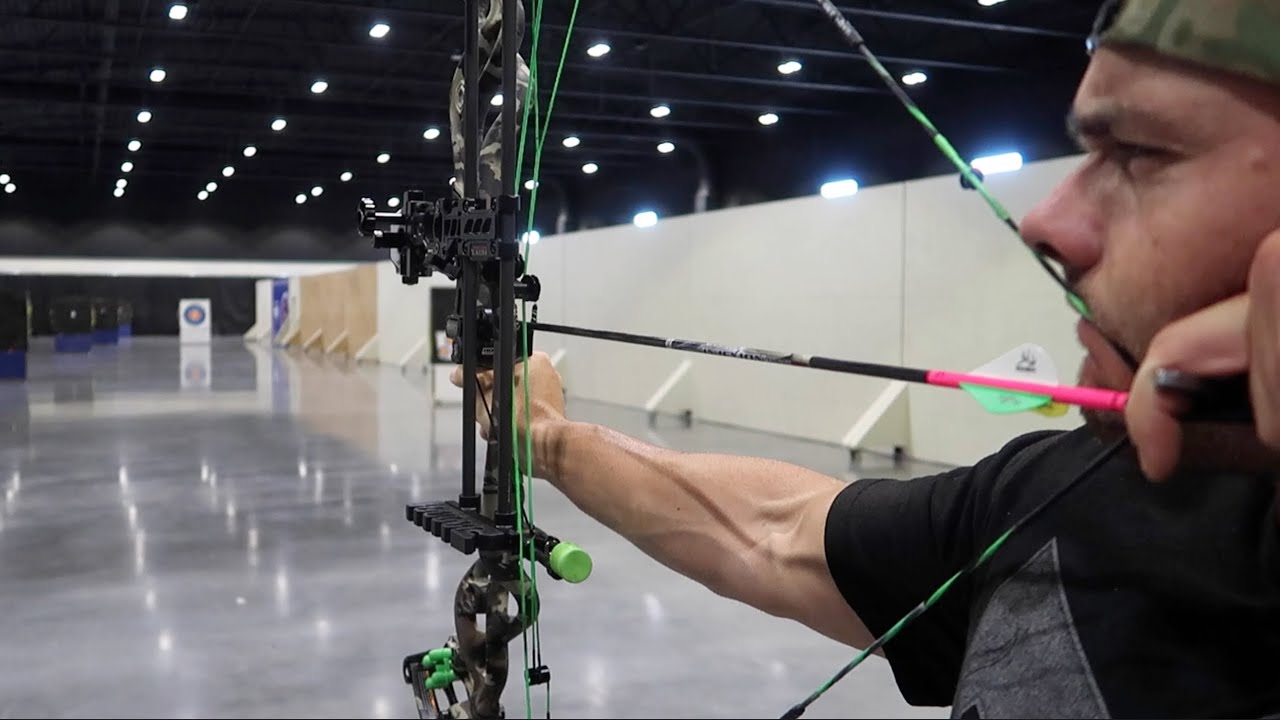This photograph captures a professional-looking Caucasian male archer at an indoor shooting range, meticulously drawing back an arrow on a hefty, modern crossbow. The man appears focused, ready to release the arrow towards a distant target, which is approximately 50 feet away. The image is taken from the left side, emphasizing his muscular build as he holds the bow with his right hand and pulls the arrow with his left. The bow is predominantly black with subtle gray and green detailing, featuring a green and black string. The arrow he has drawn is mainly black with a pink notch at the end. The surroundings of the range are utilitarian, with white walls and a grayish-black concrete or marble floor. Overhead, the warehouse-like structure is illuminated by several ceiling lights. Temporary partitions are set up along the sides for safety. The overall setting is stark and functional, focusing solely on the business of archery.